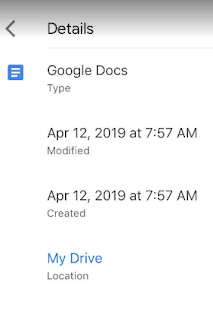This is a detailed screenshot of the information pane for a Google Doc stored in Google Drive. The pane is accessed by selecting the "Details" option from the previous menu screen within the app. At the top, the word "Details" is prominently displayed in black text against a fading gray background bar, accompanied by a leftward-pointing arrow indicating a back button.

Below the "Details" header, the type of file is identified as "Google Docs," with an icon next to it. This icon is a blue square featuring horizontal lines, symbolizing a written document. Further down, the pane provides timestamps showing both the creation and modification dates of the document. It states that the document was created and last modified on April 12, 2019, at 7:57 AM.

Lastly, the pane indicates the location of the document within Google Drive. The phrase "My Drive" is displayed in blue text, beneath which the term "Location" is mentioned, reinforcing that this Google Doc is stored in the user's main drive. All text is rendered in black, ensuring high readability against the white background of the pane.